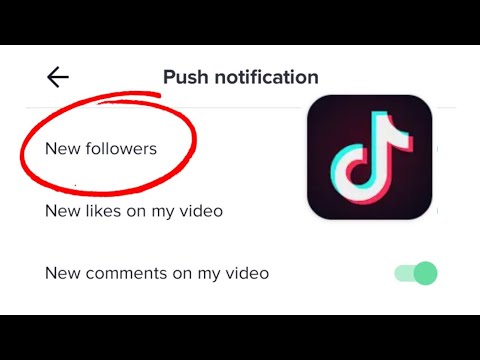The image appears to be a low-quality, out-of-focus screenshot, possibly depicting a settings menu from the TikTok app. At the top and bottom of the image, there is black text. The central portion contains various notifications and options listed in individual rows. 

On the left side, a prominent red circle highlights the 'New Followers' notification. Below, in subsequent rows, are the notifications for 'New Likes on My Video' and 'New Comments on My Video'. A green toggle switch is visible, likely indicating an option that can be enabled or disabled.

To the right of the image, the TikTok logo is present—a square icon with a musical note-like symbol in the center, displaying a blend of blue, white, and red colors. The red circle around the 'New Followers' notification nearly touches the 'New Likes on My Video' text and intersects slightly with the divider line at the top of the rows.

The pictorial content suggests the visual focus is on the notifications, particularly the 'New Followers', amidst a very pixelated background that impairs clear visibility.